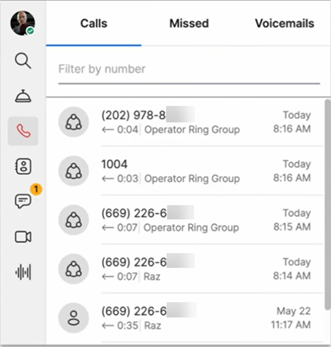**Detailed Caption of the Screenshot:**

The screenshot displays a call log interface featuring a light gray horizontal sidebar on the left side. Within this sidebar, there are various icons, including a checkmark, magnifying glass, blue icon, and a red phone icon. The sidebar also lists tabs labeled “Messages (1),” “Contacts,” “Phone,” “Video,” and “Voice.”

On the main part of the screen, a series of phone calls are listed, each marked with an icon resembling a circle with three dots. The phone calls display partial numbers, such as 202-978-1XXXX, and some specific details are shown in the call log. For instance, one entry is labeled "Operator Ring Group" with a timestamp of 8:00 AM, with subsequent calls at 8:15 AM, 8:30 AM, and further times.

Further down, there is another entry with the number 1-0-0-4-6-6-9, indicating the time of the call and additional details. The log also notes that voicemails are directed to a specific number. The last call listed occurred at 11:17 AM on May 22nd, with the rest of the calls marked "today," suggesting they are from the same day as well.